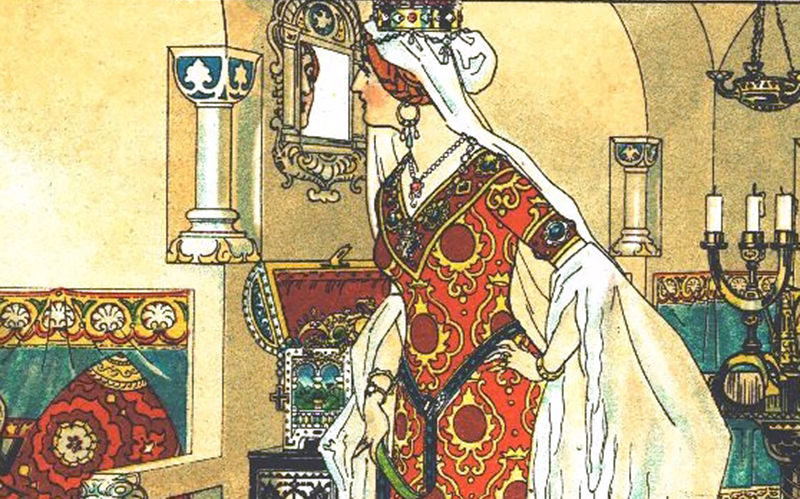This detailed, colorful illustration depicts a lavish medieval scene featuring a regal woman, possibly a queen, adorned with an array of intricate and ornate jewelry. She wears a golden crown encrusted with jewels, a long white headdress or shawl that drapes over her back, and elaborate long earrings. Her striking red dress is richly designed with elaborate yellow and black patterns, complemented by a v-neckline and adorned with gold, blue, and green accents. She also sports a beautiful necklace with a red pendant and a sash around her waist.

The setting around her exudes opulence, with beige walls decorated with little columns and pillars outlined in black. The room is filled with lush, colorful draperies in green, red, and gold, along with numerous candelabras and a chandelier. In the background, an open treasure chest spills over with a dazzling assortment of jewels and a Christian cross. This resplendent scene is accentuated by vivid background colors of blue, yellow, and red, bringing to life the emphasis on the subject's luxurious and rich surroundings.